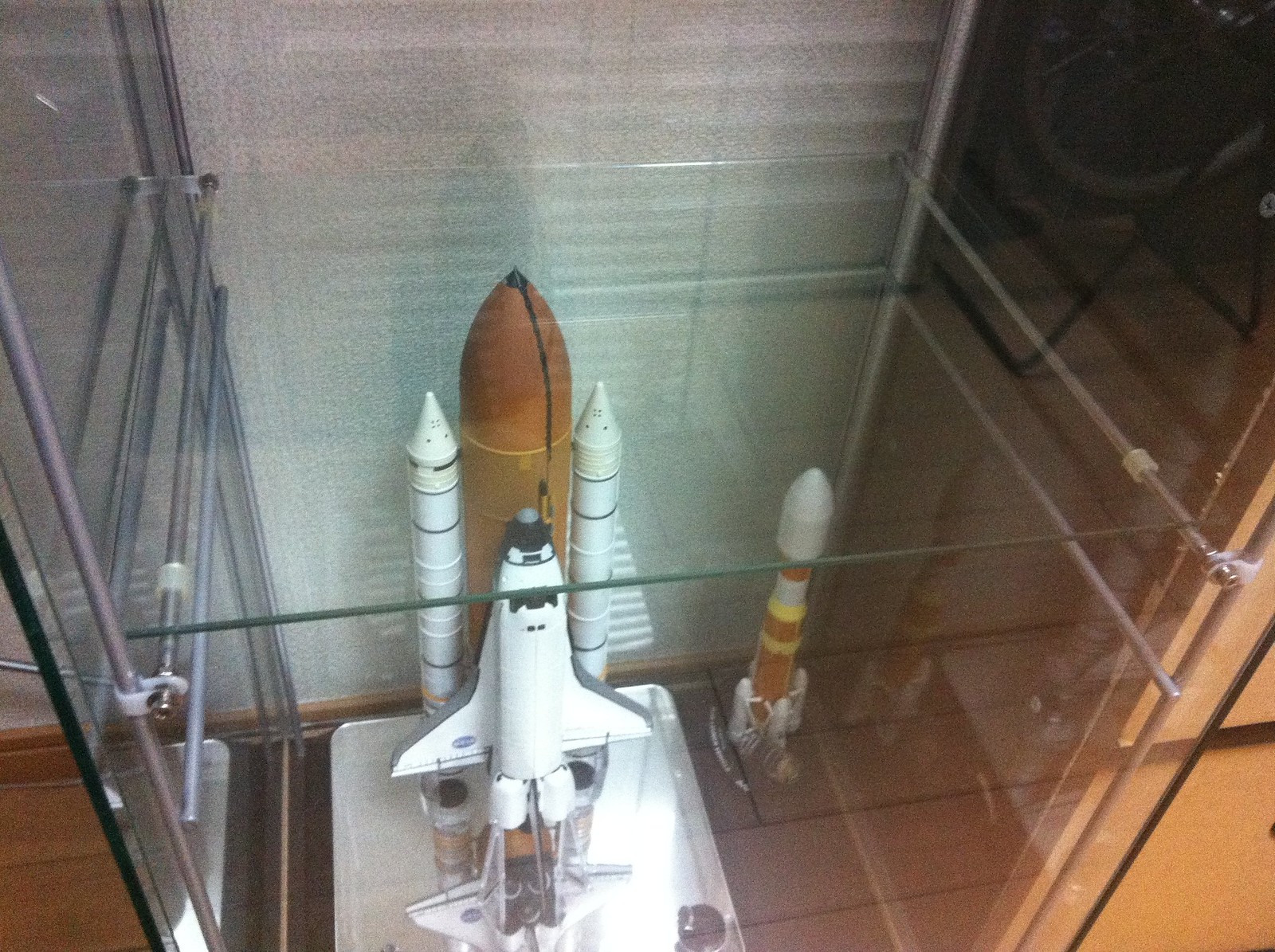This photograph, likely taken in a museum, showcases a meticulously detailed model display encased in a glass case. Central to the exhibit is a scaled-down model of a space shuttle, reminiscent of NASA's iconic spacecraft. The shuttle, painted white with gray-edged wings, is affixed to a large, bright orange booster rocket, which stands upright as if poised for launch. Flanking this booster are two supplementary white rockets, each adorned with small, metallic bands that appear to be made of brass or copper. Additionally, the display features another distinct rocket with a white tip and a red-and-yellow striped body. The entire assembly is mounted on a white platform, with a metallic plate beneath the central booster reflecting its underside. The glass case and surrounding metal bars not only protect the models but also maintain the display's structural integrity, allowing viewers to appreciate the intricate details of the miniature space exploration setup.